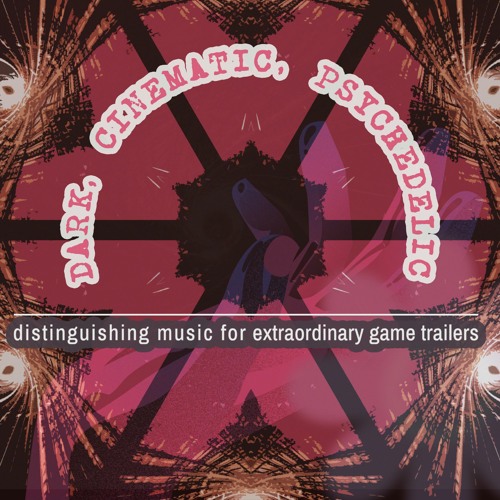The poster features a dark, dynamic theme with a predominantly dark purple background. At the center, there's an almost diamond-shaped, black figure resembling an octagon. From this shape, six straight black lines radiate outward, extending to the edges of the image. Surrounding this central shape are swirling patterns in gold and white, adding to the psychedelic aesthetic.

The text on the poster is prominently displayed in pink and white lettering. Curved across the center is the phrase "Dark, Cinematic, Psychedelic," outlined in white and further bordered in grey. Below this, there is a skinny horizontal white line. Beneath the line, more text reads, "Distinguishing Music for Extraordinary Game Trailers," also in white lettering. The combination of the vivid colors and dynamic shapes emphasizes the poster's dramatic and psychedelic theme.